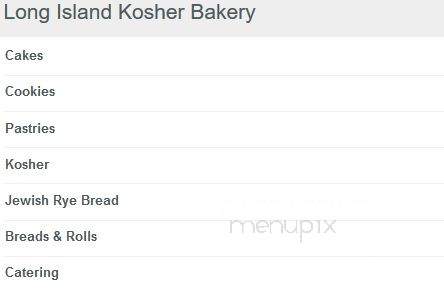The image showcases a chart from a Long Island kosher bakery. At the top, in a larger and dark gray font, the text reads "A Long Island Kosher Bakery," with each word's initial letter capitalized. This title is set against a long, grayish rectangle background.

Below the title, there is a chart listing various products offered by the bakery. The chart is segmented by gray lines, separating each product category. The categories listed are:

1. Cakes
2. Cookies
3. Pastries
4. Kosher
5. Jewish Rye Bread
6. Breads and Rolls
7. Catering

Each product category is written in gray text, with only the first letter capitalized.

In the lower right corner of the chart, there is a faint, light gray watermark in lowercase that reads "menu p1x." The entire image has a slightly low-resolution appearance.